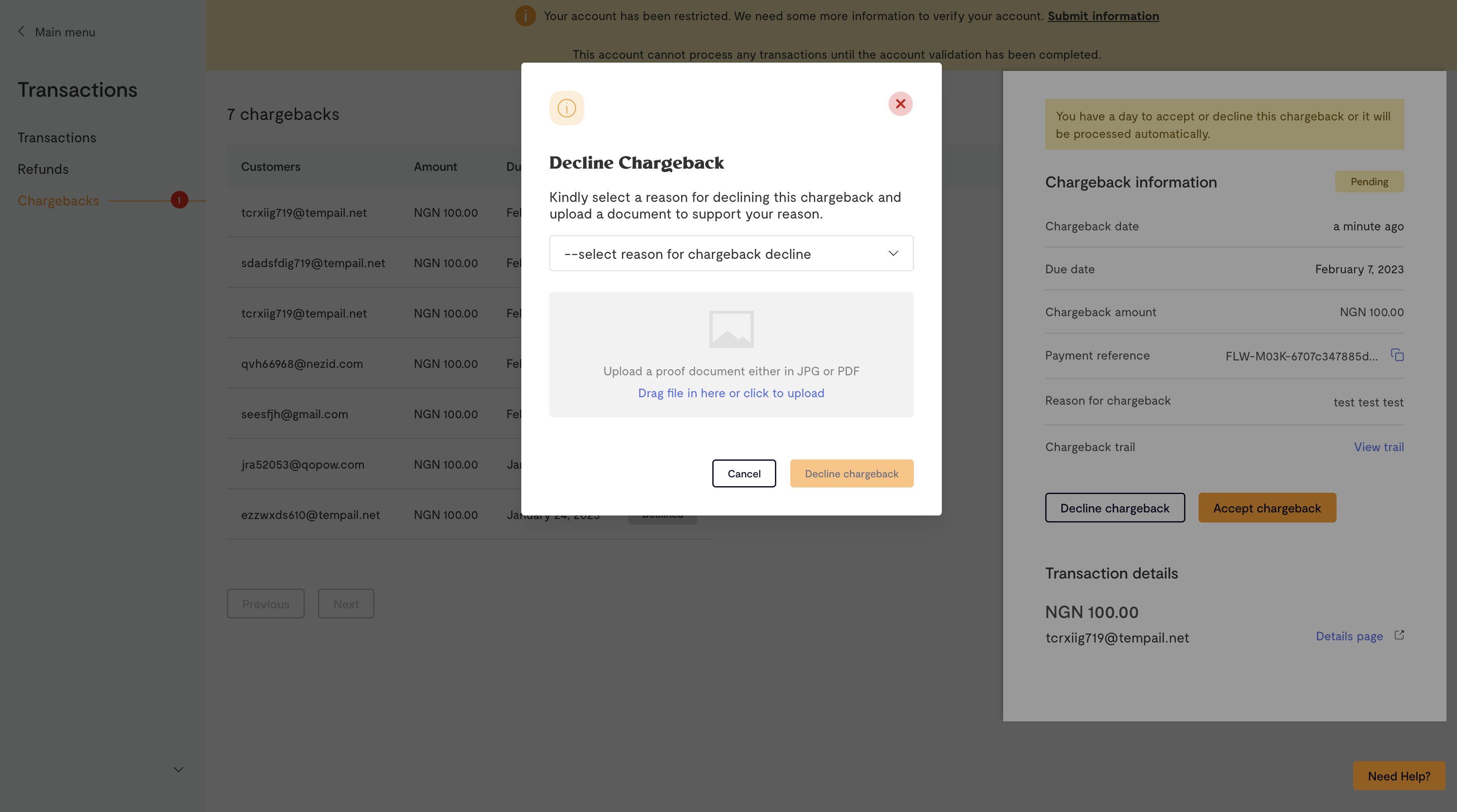The image depicts a grayed-out background featuring a partial view of transaction-related details. To the left, there are black text headings for "Transactions," "Transactions," "Refunds," and "Chargebacks," along with a list of seven chargebacks, each paired with email addresses and amounts, the full details of which are obscured by overlapping pop-ups.

In the center, a rectangular pop-up with a white background is prominently displayed. It is marked by an orange circle in the upper left corner and a red 'X' in the upper right corner. Central black text reads, "Decline Chargeback." Instructions below ask the user to "Kindly select a reason for declining this chargeback and upload a document to support your reason." Beneath this, there is a drop-down menu labeled "Select Reason for Chargeback" and an area designated for uploading evidence, which states, "Upload proof of document in either a JPEG or PDF. Drag file here or click to upload." At the bottom, two buttons offer options to either "Cancel" or "Decline Chargeback."

To the right, there's another, slightly larger rectangular pop-up. It informs the user they have one day to either accept or decline the chargeback, warning that it will be processed automatically if no action is taken. This pop-up lists chargeback information including a "Pending" status, "Chargeback Date" of a minute ago, "Due Date" of February 7, 2023, "Chargeback Amount" of NGIN 100, a "Payment Reference" number, and the "Reason for Chargeback," which here reads, "Test test test." Additional buttons at the bottom offer options to "Decline Chargeback," "Accept Chargeback," view "Transaction Details," and provide an email address for further contact.